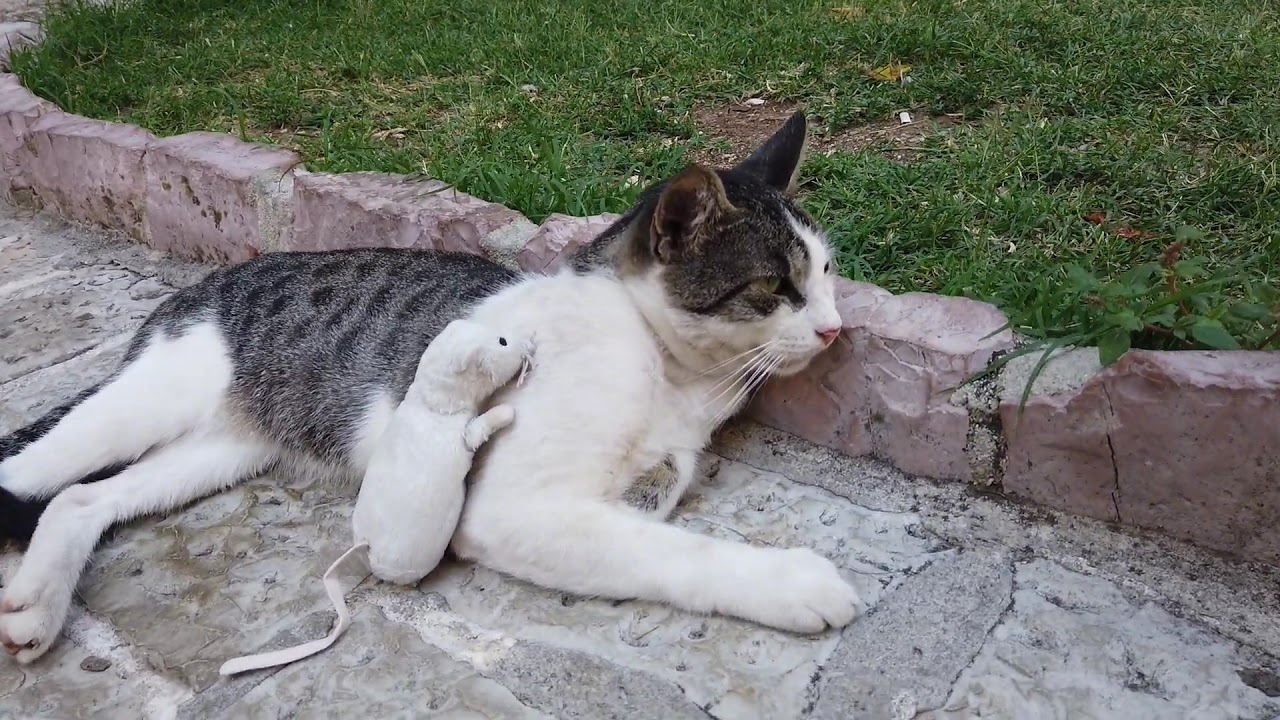A close-up image shows a lounging cat on an outdoor walkway composed of square, 8-inch wide pinkish-gray tiles with concrete filling the gaps. The walkway features an edge or guard on the side, beyond which patchy green grass can be seen. The cat, which is predominantly white with dark gray and black spots reminiscent of a cheetah, has its head resting on the edge of the walkway. Its right side, including the shoulder, supports a white toy mouse with a matching tail. The cat’s face is a mix of black and white, particularly on one half, and it has a long, spotted tail. The feline appears relaxed, looking slightly to the left with its ears perked up, suggesting a serene moment on a sunny day.